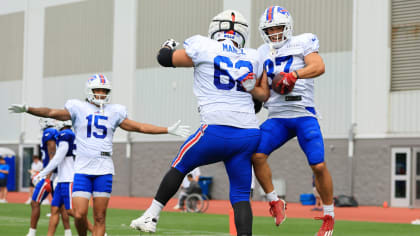This vibrant landscape photograph captures a group of five young football players during a practice session on a green field, likely at a high school or college. The athletes are energetically jumping around, perhaps engaged in calisthenics or dancing, with some appearing to be in mid-air. They are all dressed in bright blue shorts, some with an orange stripe down the side, and white short-sleeved shirts with royal blue numbers—prominently featuring numbers 62, 15, and 87. The main player in the forefront, donning a shirt with the bright number 62 and the letters "MA" or "N" visible on the back, stands out. Another player to his right, with a light-skinned face and a broad smile visible through his helmet, gazes directly at the camera. His helmet is white with a distinctive light blue and red stripe down the center and a blue circle with a red stripe on the side; he holds a red ball in his gloved right hand. The background of the image features a gray and white industrial-looking building that resembles a school, a possible stadium, and additional players dressed in varying gear. One notable detail includes a gentleman in a wheelchair, implying inclusivity and support within the team environment. The overall scene depicts a lively, cheerful atmosphere amidst the youthful team's training session.